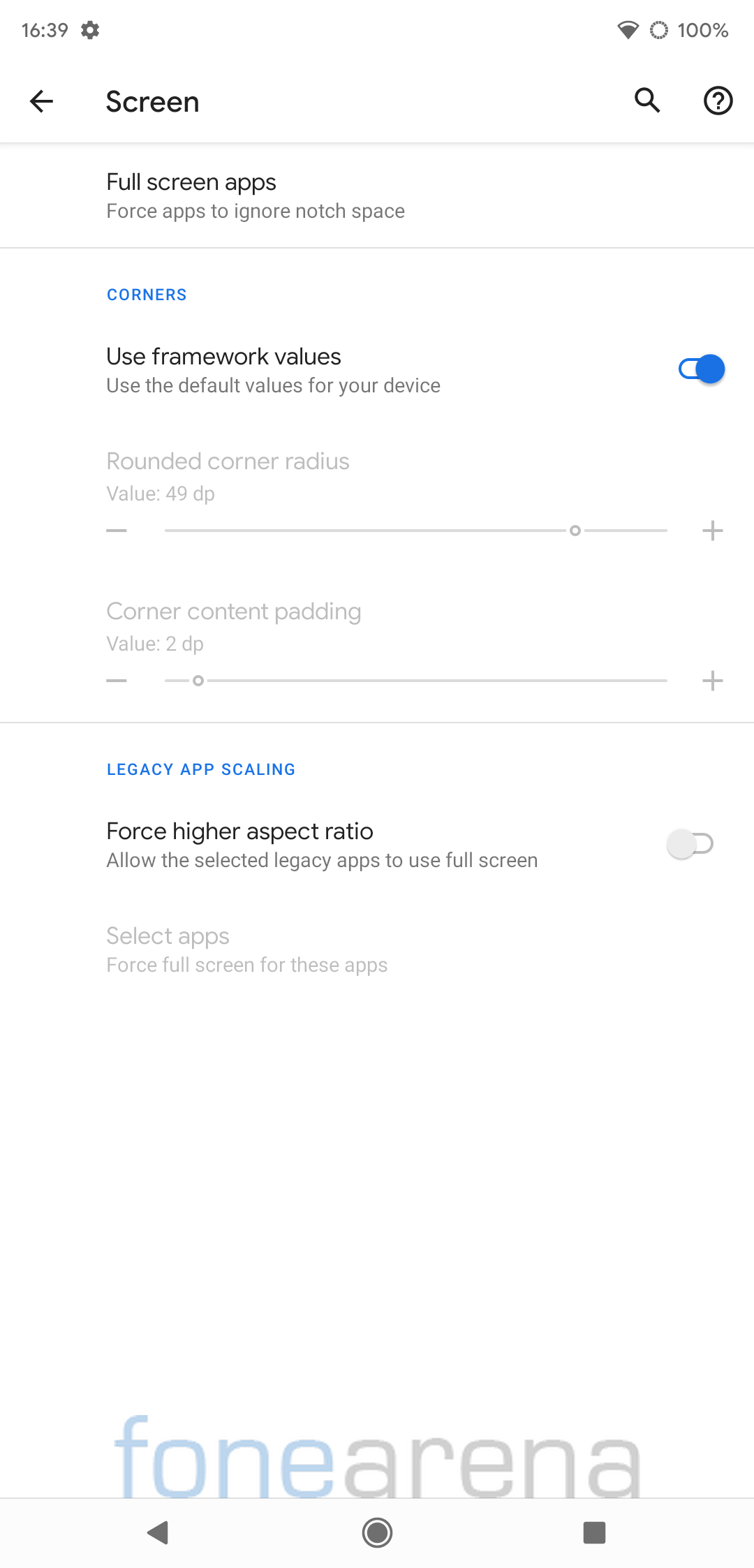Screenshot of a cell phone screen displaying the settings interface:

- **Top Bar:**
  - **Left:** Time is displayed as 16:39, accompanied by a settings icon.
  - **Right:** Battery indicator shows 100% charge.

- **Main Interface:**
  - **Header:** Contains a left arrow labeled "Screen" with icons for search and a help bubble (question mark) on the right.
  - **Section Header:** "Full Screen Apps"
    - **Description:** "Force apps to ignore notch space"
    
  - **Divider Line**

  - **Settings Section:**
    - **Label:** "Corners" (in blue, all caps, small font)
    - **Option:** "Use framework values" (in black font)
      - **Description:** "Use the default values for your device" (in smaller font)
    - **Control:** A selection option on the right, depicted as a blue toggle.
    - **Label:** "Rounded corner radius" (in lighter gray font)
    - **Value:** "Value 49 dp" with a line and a plus sign to the right.
  
  - **Divider Line**
    
  - **Next Setting:**
    - **Label:** "Corner content padding"
    - **Value:** "Value 2 dp" with another line and a plus sign.

  - **Divider Line**

  - **Section Header:** "Legacy App Scaling" (in blue, all caps)
    - **Option:** "Force higher aspect ratio"
      - **Description:** "Allow the selected legacy apps to use full screen" 
    - **Control:** A gray button to the left indicating the option is off.
    - **Option:** "Select Apps"
      - **Description:** "Force fullscreen for these apps"
  
  - **Footer:**
    - **Label:** "FONE" (in blue)
    - **Label:** "arena" (in gray)
  
  - **Navigation Bar:**
    - **Icons (Left to Right):** Left arrow, central button, black square.